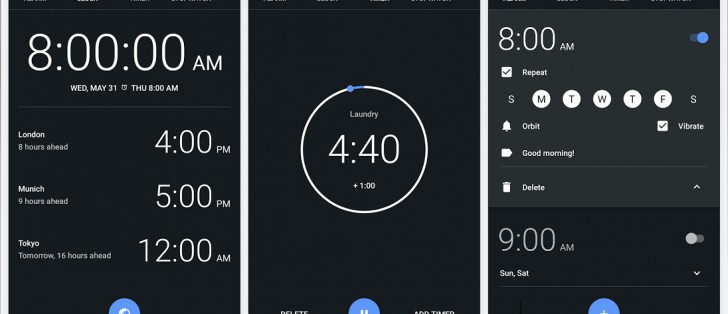The image is a composite screenshot consisting of three individual screenshots placed side by side. Each screenshot features a solid black background with white text, displaying different types of information.

The first screenshot shows a list of global times and dates:
- "8 a.m. Wednesday, May 31st"
- "Thursday, 8 a.m."
- "London: 8 hours ahead, 4 p.m."
- "Munich: 9 hours ahead, 5 p.m."
- "Tokyo: tomorrow, 16 hours ahead, 12 a.m."

The second screenshot features a round white circle with the text "laundry" and "440+1" inside it. Below this circle, there are buttons labeled "Delete" and "Add Timer."

The third screenshot displays a time, "8 a.m.," along with a weekly calendar layout labeled "Sunday to Saturday." Additional elements in this screenshot include the greetings "good morning," a delete icon, and a check mark next to the word "vibrate."